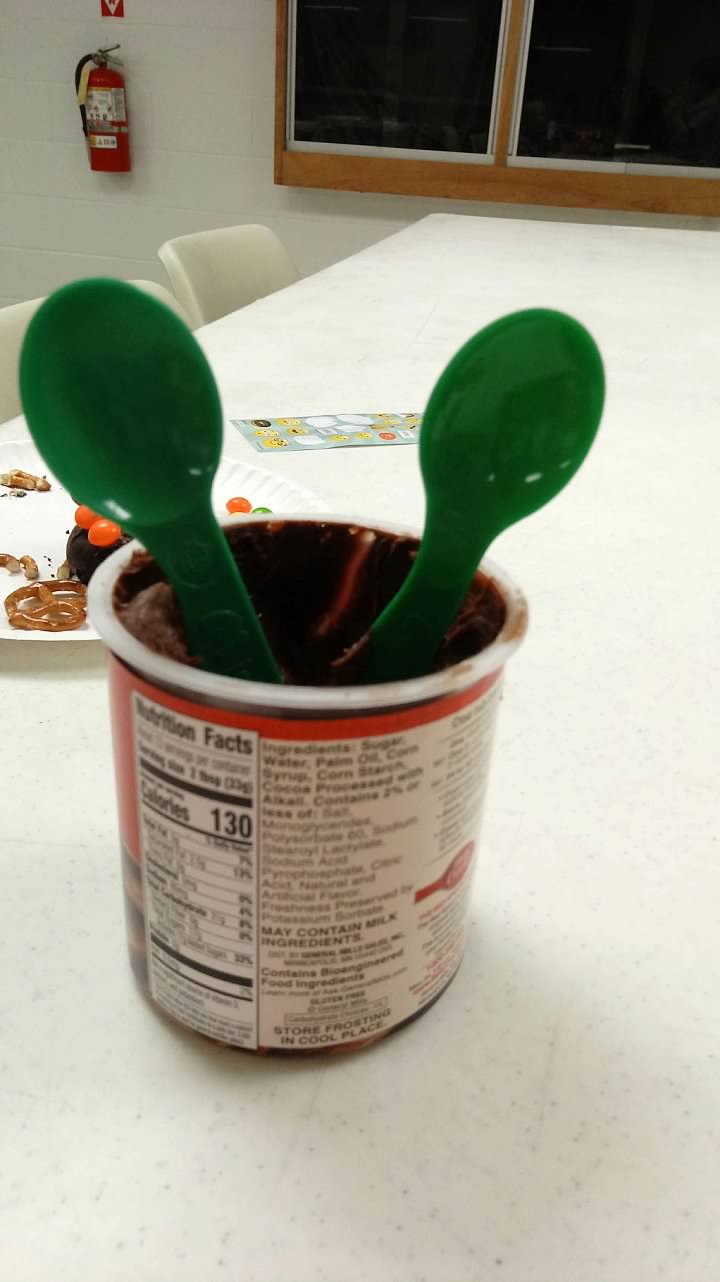This photograph features an open tub of Betty Crocker chocolate frosting prominently placed in the center on a white countertop. Two green plastic spoons are inserted upside-down into the frosting, implying someone might scoop some out directly. Behind the tub on the same white counter is a paper plate laden with a mix of pretzels, brownies, and M&Ms. The backdrop includes a stark white cinder block wall, a mounted red fire extinguisher, and a set of windows framed in wood on the right, through which the dark outside contrasts with the brightly lit interior. White chairs are also visible around the scene, contributing to the overall bright and clean ambiance.